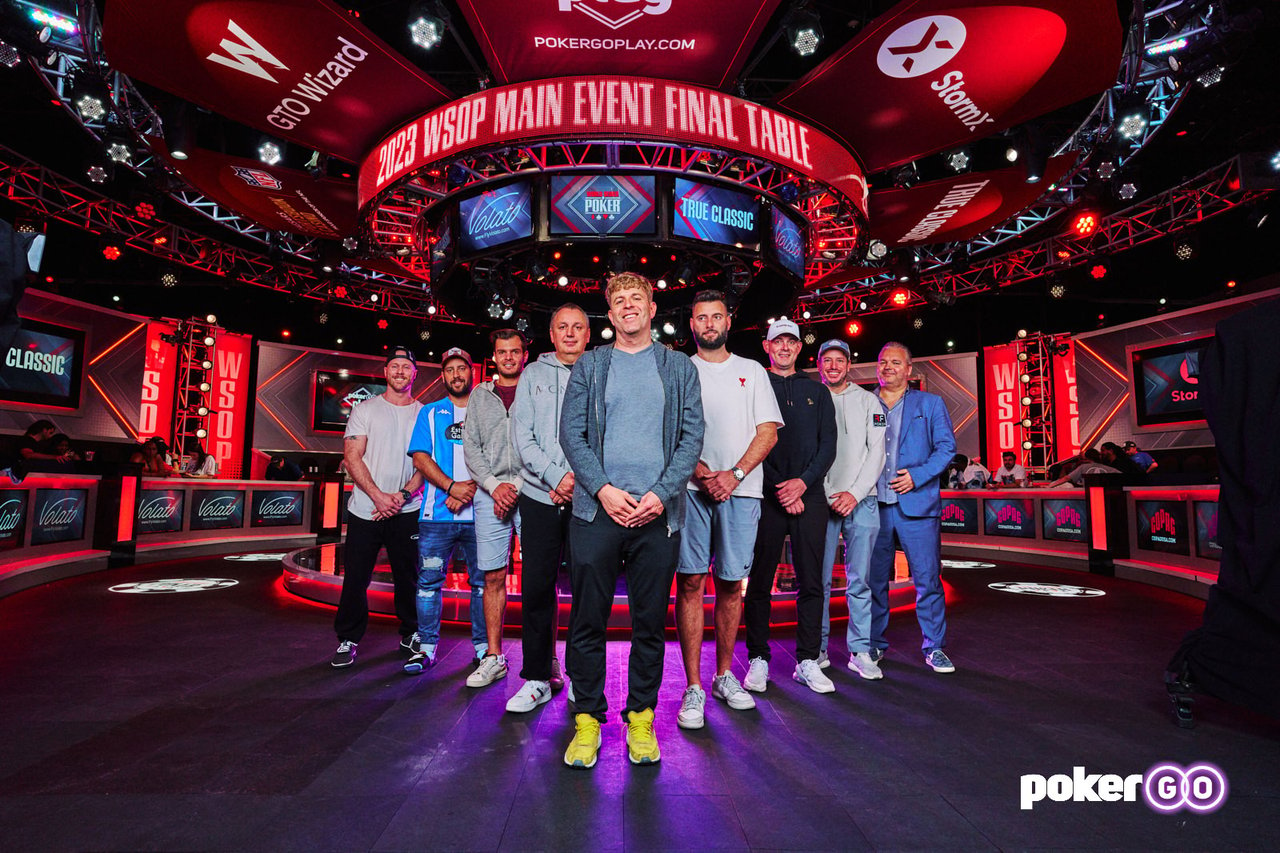This photograph captures nine white male participants of the 2023 World Series of Poker (WSOP) Main Event Final Table, organized in a reverse horseshoe or V formation, facing the camera. The men are casually dressed, sporting t-shirts, hoodies, shorts, sweatpants, and various sneakers—including a notable pair of bright yellow sneakers worn by the man in front. The background features a series of video screens and a prominent banner reading "2023 WSOP Main Event Final Table." The set is primarily illuminated by red lights, creating a dark yet vibrant atmosphere, with the floor appearing purple. Corporate logos for GTO Wizard, PokerGoPlay.com, and StormX are also displayed above the participants. In the bottom right corner, the Poker Go logo is visible.